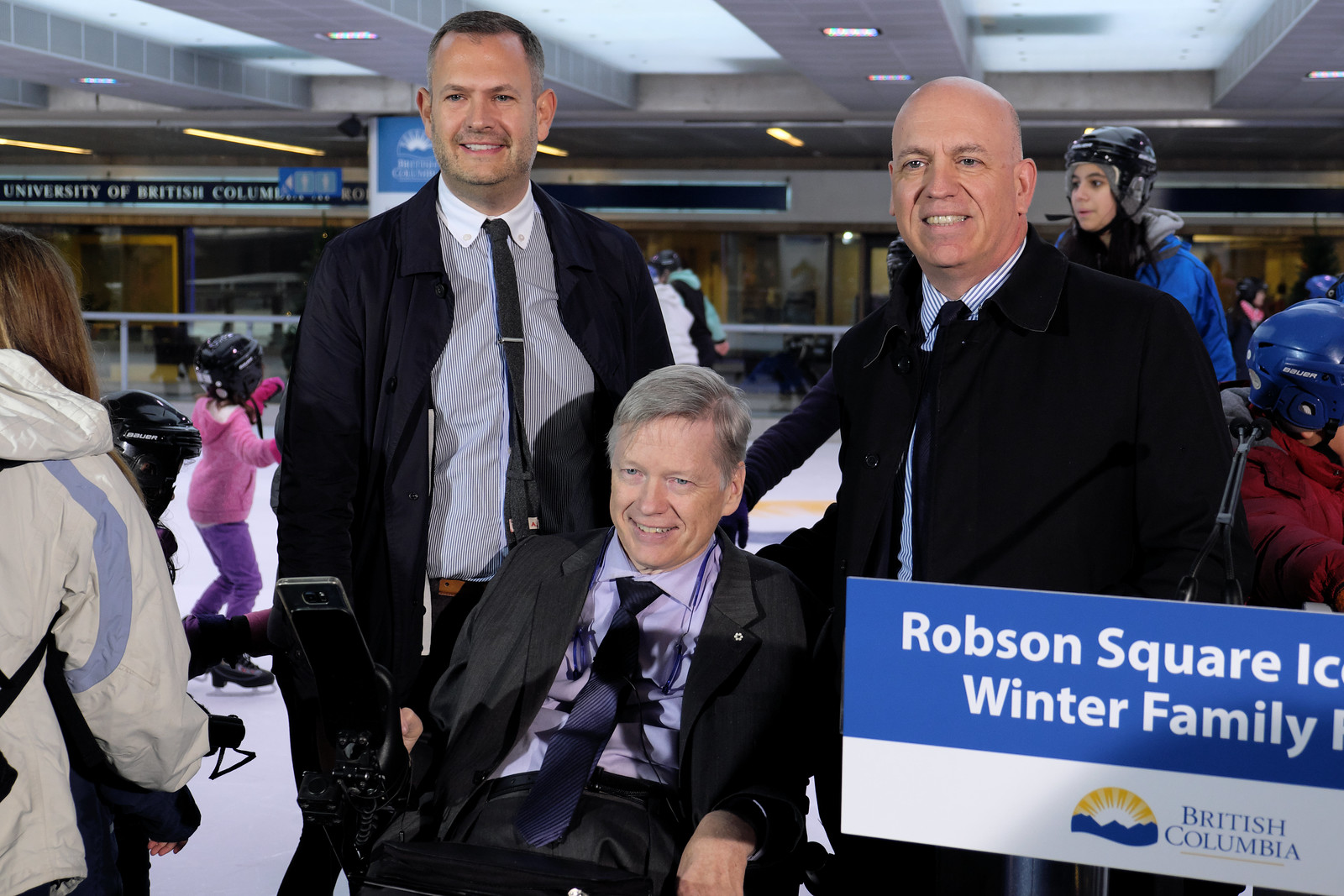This image captures a vibrant scene at an indoor ice skating rink, identified by signs reading "University of British Columbia" and "Robson Square Ice Winter Family" in blue and white lettering. Dominating the foreground are three men in the 35-40 age range, with the man in the middle sitting in a wheelchair, dressed in a suit with a purple shirt and tie. Flanking him are two smiling men in suits; the man to the left (from the viewer's perspective) wears a white shirt with a thin tie and a dark blue jacket, while the man to the right, who is bald, sports a purple shirt. The bald man has his arm gently resting behind the man in the wheelchair. In the background, on the left, a young girl about five to seven years old is visible ice skating, donning a pink shirt, pink coat, purple pants, and a helmet. To the right, a few other individuals are seen skating, including some wearing crash helmets. The scene is lively and appears to be a family event, with the ice rink featuring a white ceiling with lights descending from it.